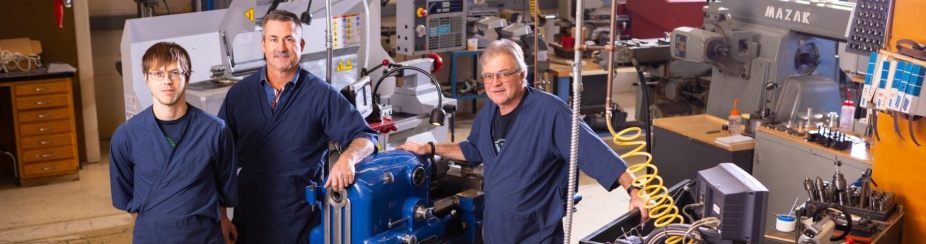In this photograph set in a bustling, cluttered workshop, three light-skinned men stand in a line, all clad in simple blue kimono-like robes over plain clothing. The men's ages appear to span three generations: a younger man in his 20s, a middle-aged man in his 40s or 50s, and an older man perhaps 20 years senior. The workshop around them is filled with mechanical and electrical equipment, including a central blue machine that resembles an engine, a yellow pneumatic hose, a variety of tools, and what appears to be a MAZAK machine, partially visible with its letters in the top right corner. The workspace features numerous drawers with gold handles, a dark orange section in the top right corner, and a light tan tiled floor. The men’s attire, the mechanical environment, and familial appearance suggest they are likely part of a family-run business, perhaps pictured here for an “About Us” section on their company’s website.